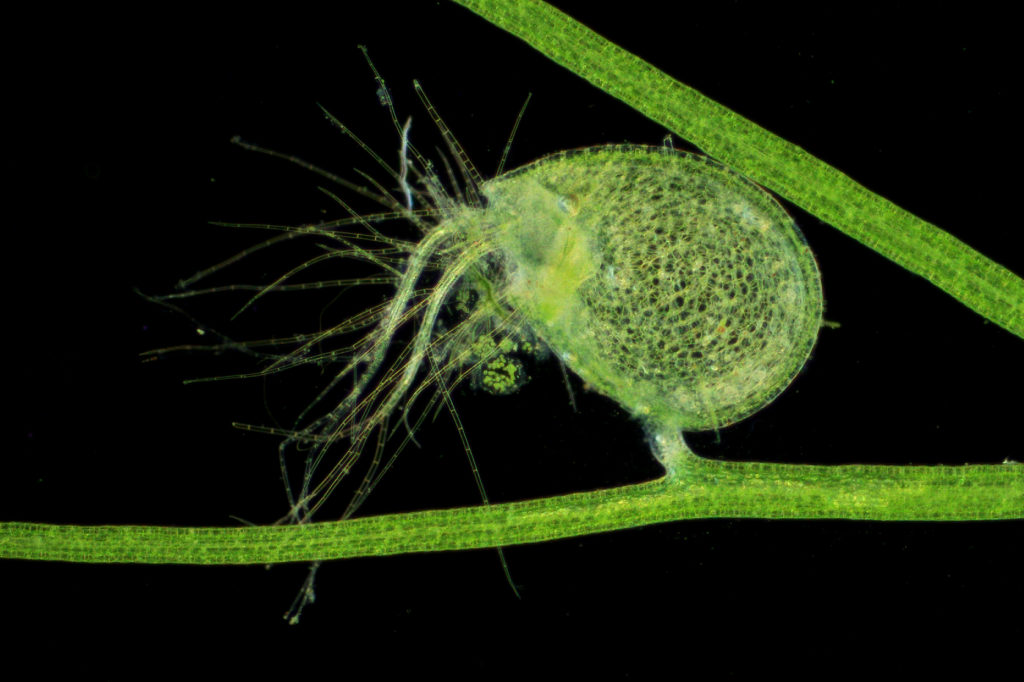This highly detailed microscopic photograph showcases two distinct green stems with intricate cellular structures, set against a stark black background. The first stem originates from the right side of the image and sharply angles upward, disappearing off the top edge. The second, lower stem extends horizontally across the entire frame from left to right. Centrally positioned on the lower horizontal stem is a prominent, circular structure resembling a plant sprout or bulbous appendage. This structure is densely packed with dark cellular formations and features a translucent appearance with varying densities. From its left side emanates a burst of approximately thirty filament-like protrusions, reminiscent of tendrils or tentacles, suggesting an explosive, dynamic growth. The vivid green and yellow hues within the structures contrast sharply with the dark backdrop, highlighting the intricate complexity and mystery of the subject, which intriguingly blurs the line between plant and animal characteristics.